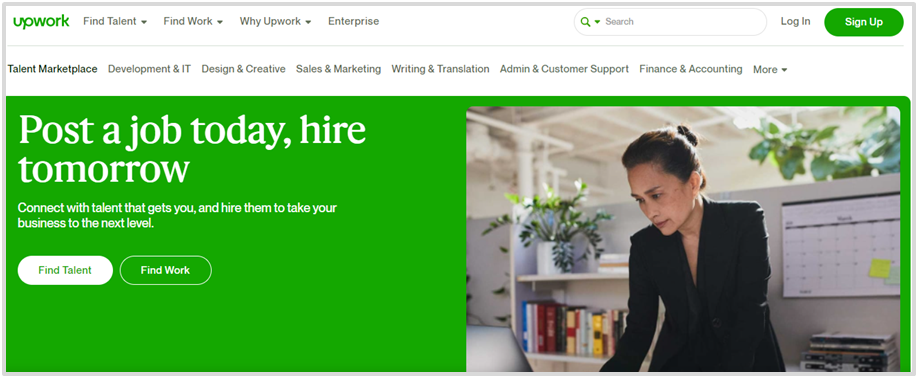The image displays a homepage of Upwork, with a primary focus on its interface for connecting employers with freelancers. Dominating the scene is the company's name, "Upwork," highlighted in green. Key sections include "Find Talent," "Find Work," "Y Upwork," and "Enterprise." 

At the top, a search bar features a green magnifying glass icon, suggesting ease of navigation. To the right, a green oval button reads "Log In," and a contrasting white "Sign Up" text is inscribed on another green oval. 

The main navigation menu presents categories labeled in a clear, bold font: Talent Marketplace, Development & IT, Design & Creative, Sales & Marketing, Writing & Translation, Admin & Customer Support, Finance & Accounting, and More. Notably, "Talent Marketplace" is emphasized in bold.

A central visual depicts a professional woman in a black suit, seated within an office-like cubicle, her hair neatly arranged in a bun, exuding professionalism and readiness. 

Adjacent to her image, on the left, is a green square with a motivational prompt: "Post a Job Today, Hire Tomorrow. Connect with talent that gets you and hire them to take your business to the next level." Below this, a white oval button displays "Find Talent" in green text, and a green oval button reads "Find Work" in white, offering clear paths for employers and job seekers alike.